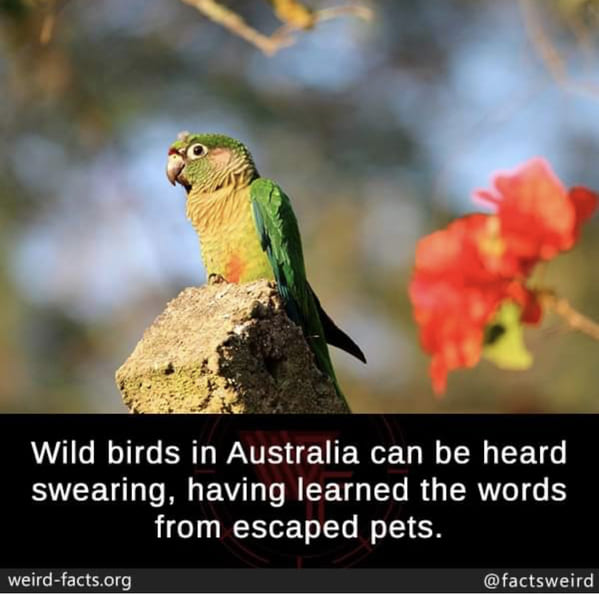The image showcases a small, exotic parakeet-like bird with striking colors. The bird predominantly features green plumage, with a pale tan or pink hue on its cheeks. Its eyes are marked with black and white patterns, and its beak is primarily grayish-brown, accented with a touch of red near the base. The bird's belly transitions into a yellowish-green shade. It is perched delicately on one edge of a rectangular stone. The background is artistically blurred, creating a bokeh effect, and reveals hints of branches and a vivid red and green flower situated to the right of the bird. 

The lower half of the image contains a black text box with white lettering, displaying an intriguing fact: "Wild birds in Australia can be heard swearing, having learned the words from escaped pets." This text is accompanied by a logo and additional text, with the logo for weirdfacts.org located at the bottom left and the Twitter handle "@FactsWeird" positioned at the bottom right. The background framing this information is primarily black with red accents.